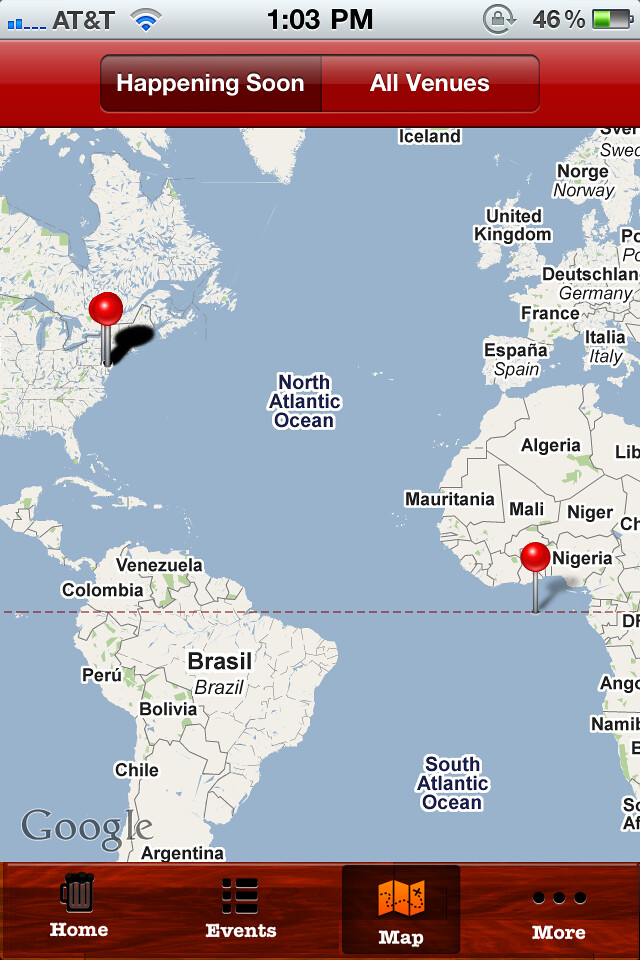This image captures a screenshot of a world map from a smartphone, highlighting significant event locations under the prompt "Happening Soon." The map showcases continents including North and South America, segments of the Atlantic Ocean, Europe, and Africa. The top of the screen displays typical smartphone interface elements, indicating the service provider AT&T, the time as 1:03 p.m., and a battery level at 46%. Notably, the map features prominent red pins marking two distinct locations: one within a New England state in the U.S., and another near the equator, just beneath Nigeria. Despite the markers, the specific event details remain undisclosed.